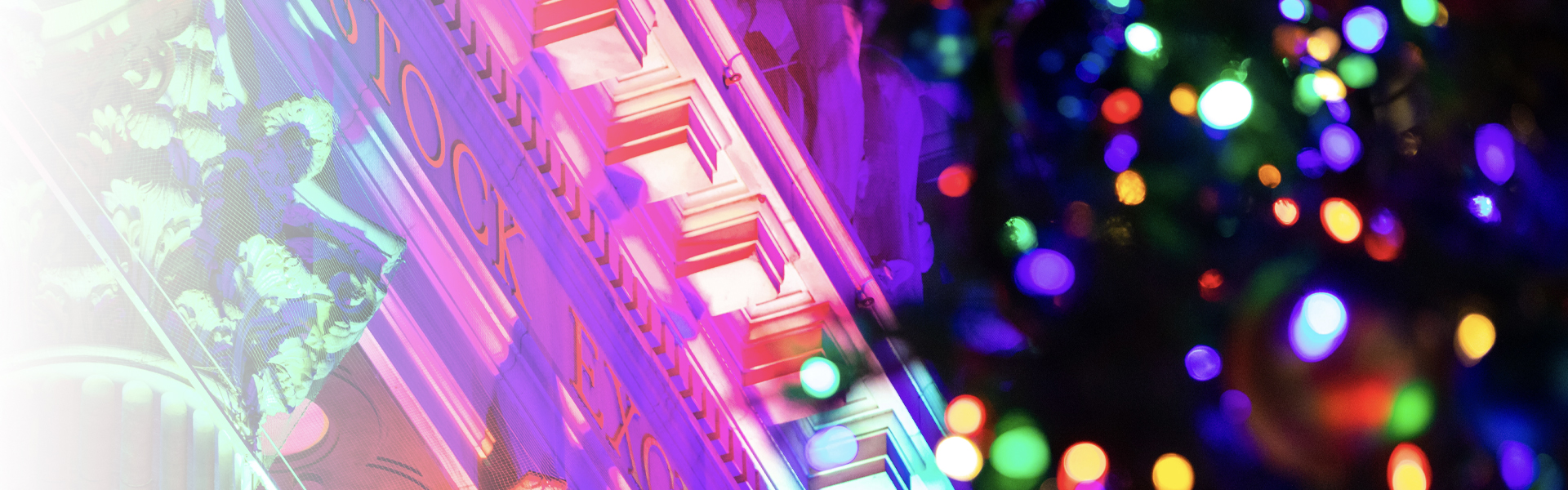The image is a wide, thin banner graphic that depicts a nighttime scene. The left side of the image reveals part of a building with architectural features resembling a Greek Revival structure, potentially a depiction of the New York Stock Exchange. The building is illuminated with neon lights in shades of teal, pink, and purple. The visible signage on the building reads "Stock EXC," suggesting it spells out "Stock Exchange." Above the signage, there appears to be a relief sculpture. On the right side of the image, the space is predominantly black, scattered with blurry, multi-colored lights resembling Christmas lights, adding to the surreal ambiance of the scene. The lighting and gradients within the image create a mysterious and almost dreamlike quality, making it difficult to discern if the image is a real photograph or a 3D rendering.